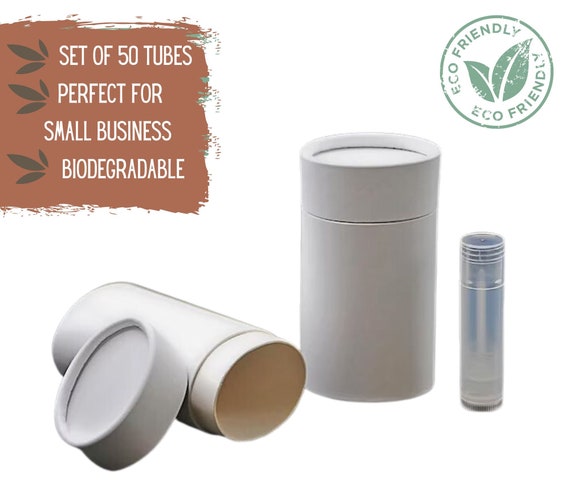The photograph is an advertisement showcasing a set of biodegradable tubes, perfect for small businesses. The image prominently features two white, non-transparent cylindrical tubes about three inches tall, made of what appears to be a cardboard material. The central tube is upright with visible lines around its upper fourth, indicating a removable cap. Next to it, another identical tube is tilted on its side with its cap off, revealing the hollow interior. To the right of these, a smaller, semi-opaque plastic tube, about one-fourth the width and three-fourths the height of the larger tubes, is also visible.

In the upper left corner of the image, against a brown background with white text and leaf bullet points, there's a label that reads "Set of 50 tubes, perfect for small business, biodegradable." Meanwhile, the top right corner features a green stamp with an eco-friendly logo showcasing two conjoined leaves. This detailed layout underscores the eco-conscious and practical nature of the product, making it ideal for environmentally aware businesses.